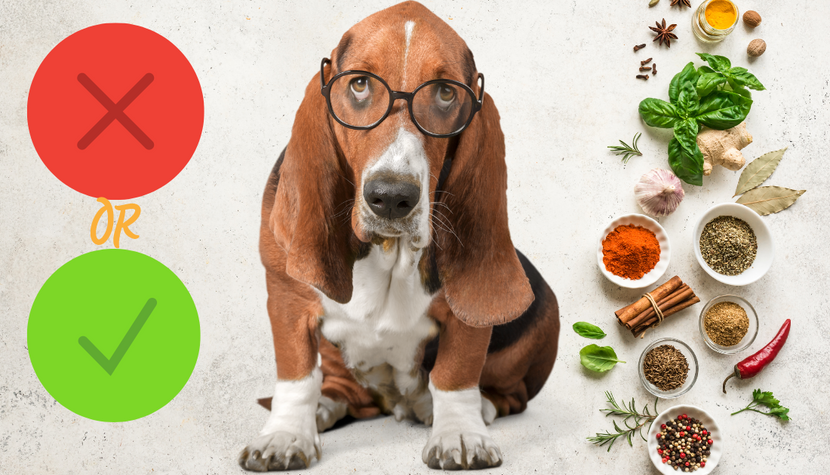In the center of the image is a hound dog with brown and white fur, sitting on its back legs and wearing large, round black glasses that give it a distinguished, almost disapproving look. To the left of the dog, there is a red circle with an X in the middle, followed by the word "OR" in an orange-yellow color, and below that, a green circle with a check mark. To the right of the dog, a variety of foods are arranged, including a display of both loose items and those in dishes. These items include an anise star, cloves, green leaves, ginger, nuts, an onion flanked by two bay leaves, and two white dishes containing green and red spices. Below these are cinnamon sticks tied with string, additional spices in three more dishes, peppers, and various leafy herbs. The overall scene suggests what foods are good or bad for the dog, creating a humorous and detailed tableau with the dog at its center, appearing like a wise, spectacle-wearing judge of culinary choices.